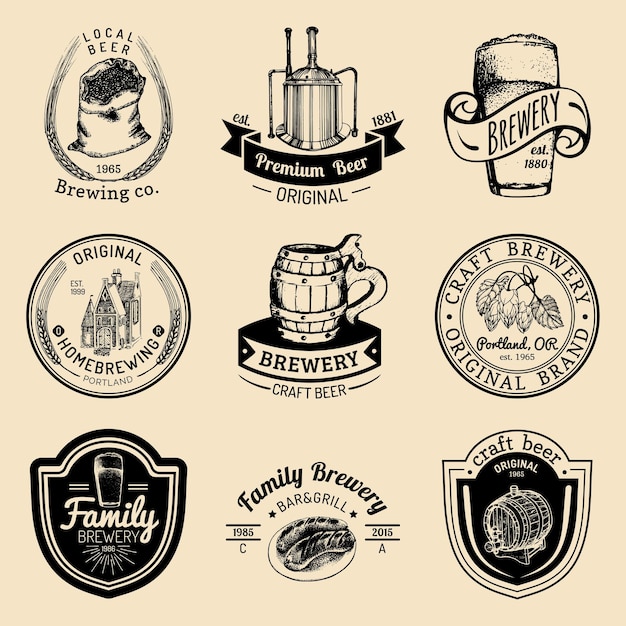The image is a detailed illustration featuring a 3x3 grid of distinct beer brand logos, presented on a cream-colored background. Each logo is intricately designed in black ink and showcases unique symbols and text representing various beer companies. 

In the top-left corner, a logo depicts a bag of barley encircled by a horseshoe of wheat, with the text "Local Beer" above and "1855 Burning Company" below. To its right, another logo features a metal tin container with a long neck, labeled "Premium Beer" and "Established 1881" on a banner. The third logo in the top row shows a glass of beer with frothy studs at the top, adorned with a ribbon that reads "Brewery, Established 1880."

In the center, the logo highlights a wooden barrel atop a platform, with a ribbon embedded in the side of the platform. This ribbon notes "Brewery" and "Craft Beer" beneath it. Additional logos, all similarly themed with references to wheat, barrels, and classic brewery imagery, fill out the remaining squares in the design. This cohesive collection of vintage-inspired beer labels captures a nostalgic and artisanal essence, making it a compelling piece of artwork or an advertisement for multiple beer brands.